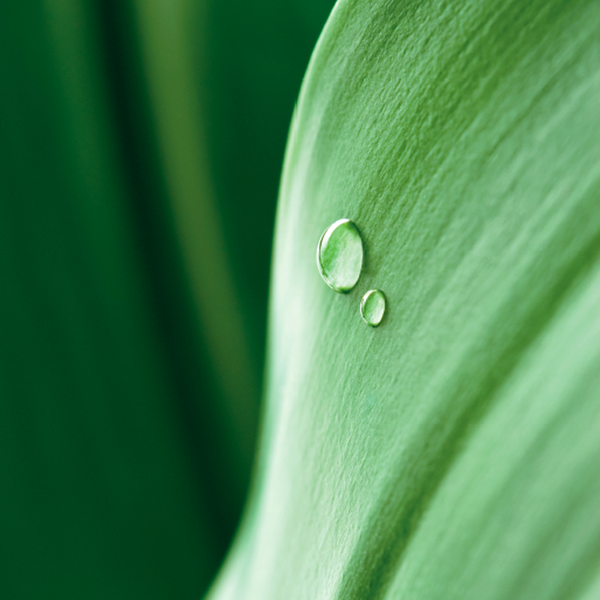The image captures a bright daytime outdoor scene, primarily dominated by shades of green. The foreground features a close-up of a plant leaf, exhibiting a soft, light green hue. On the upper middle-right part of the leaf, there are two distinct water droplets: a larger droplet positioned centrally and a smaller one to its right, both having perfect circular shapes with oval tops, gently resting on the leaf. Meanwhile, the background transitions from dark to lighter shades of green, creating a beautiful gradient effect that becomes blurred as it extends outward, providing a contrasting backdrop to the sharply focused leaf and water droplets. The overall scene lacks any text or additional moisture, emphasizing the simplicity and serenity of the natural elements captured.